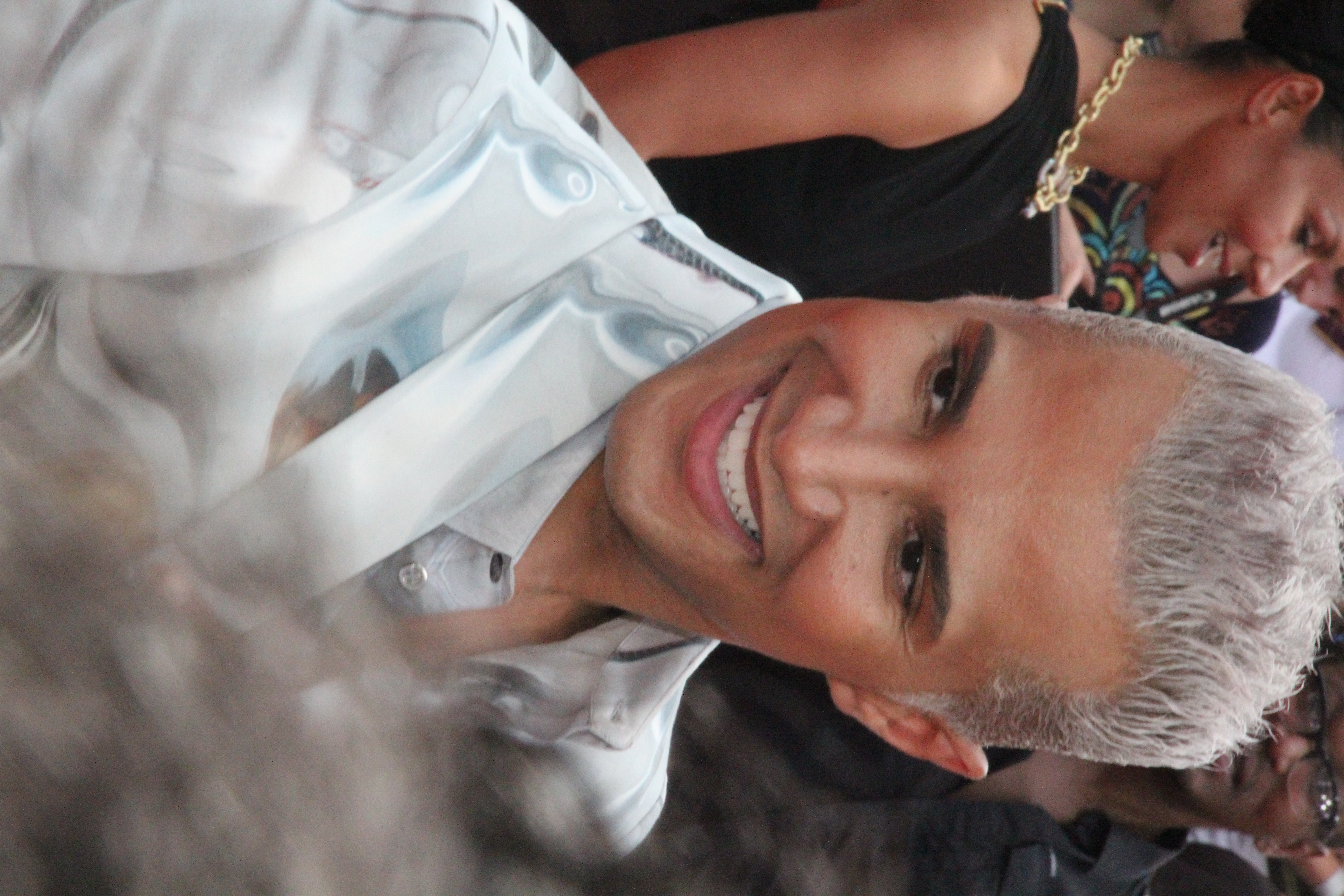This outdoor photographic image, rotated 90 degrees clockwise, prominently features an androgynous person with short, combed-up grey hair. This central figure, who could be either a man or a woman, is beaming with a broad smile, showcasing many white teeth. The individual is dressed in an eye-catching grey shirt adorned with artistic blue curved elements and has the top buttons undone.

In the background and to the left is a woman, likely Hispanic, with brown skin. She is dressed in a black sleeveless dress and wears a large chain-link necklace. She is looking slightly downward and smiling gently.

To the right and behind the central figure is a man with dark skin wearing a black button-down shirt, also unbuttoned at the top, and sporting sunglasses. In the lower left corner of the image, a slightly out-of-focus head partially obscures the view.

Overall, the photograph highlights the smiling faces and distinctive fashion choices of the individuals, creating a dynamic and lively scene.